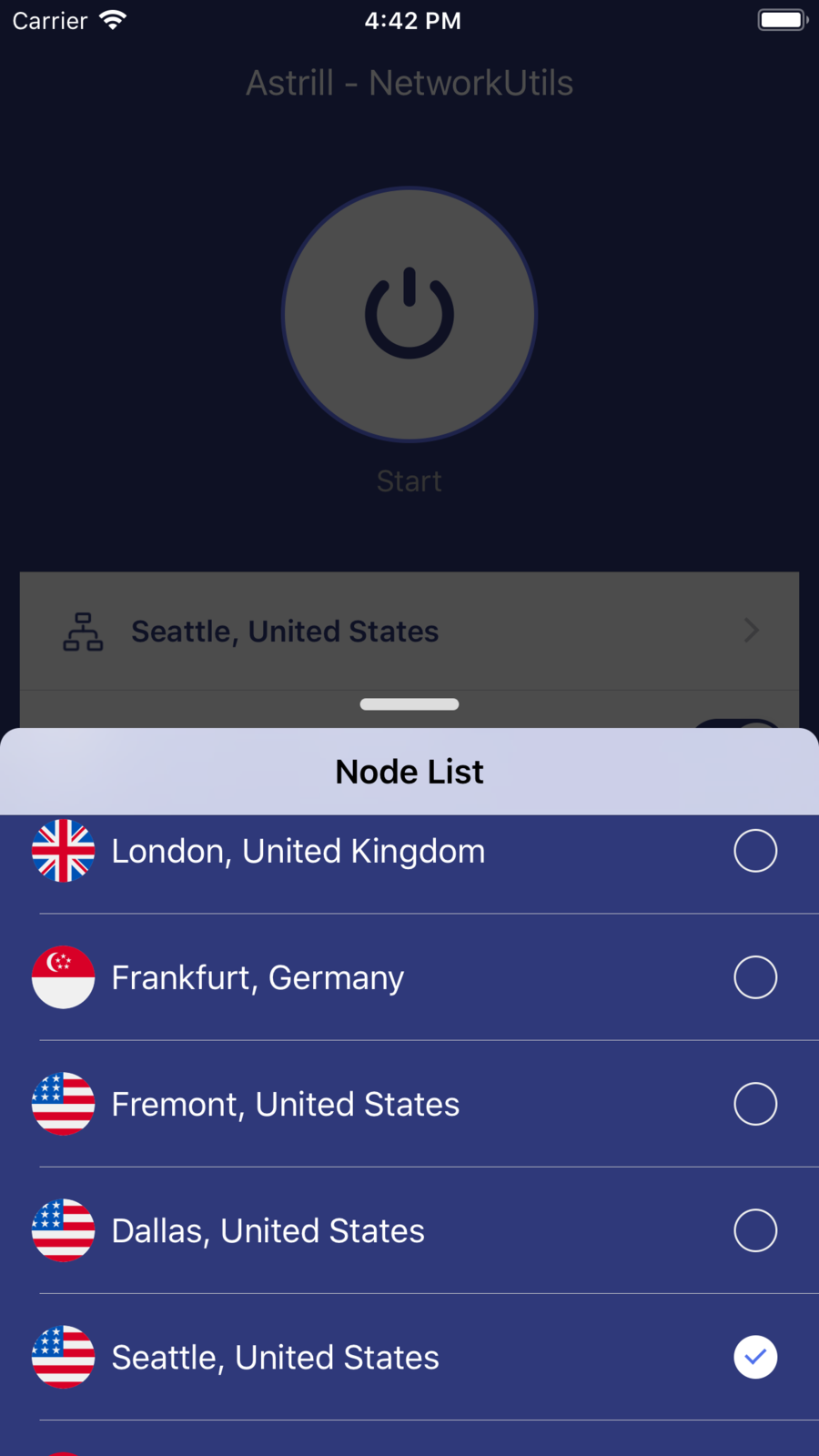The image showcases the settings screen of a mobile application against a black background with white text and icons. At the top left, there is a 'carrier' label accompanied by signal strength icons, all in white. Centrally, the time is displayed as '4:42 PM' in white text. On the top right, a white outline of a battery icon is visible. Below the time, in gray text, it reads "Astro-Network, U-T-I-L-S."

The main focus below this top section features a large white circle outlined in blue. Within this circle, there is a three-quarter open circle at the top with a thick white line. Directly underneath this symbol, the word "Start" is written, suggesting it might be a play or launch button for a feature.

Beneath this, there is a light gray banner displaying "Seattle, United States" with an arrow pointing to the right. Following this, a thin line divides the sections. The bottom portion of the image contains a white banner at the top that states "Node List" in black text. Below are five listed locations against a navy blue background, each separated by fine gray lines and accompanied by a selectable circle on the right. The locations are: 

1. **London, United Kingdom** - Accompanied by the red, white, and blue UK flag.
2. **Frankfurt, Germany** - Displaying a flag that is red at the top and bottom, white in the middle, with a moon sliver and small white stars on the red section.
3. **Fremont, United States** - Accompanied by the red, white, and blue US flag.
4. **Dallas, United States** - Also displaying the US flag.
5. **Seattle, United States** - Accompanied by the US flag and marked with a checked circle filled with white and a blue checkmark.

Another item appears to be partially visible at the bottom, showing just a hint of red, indicating that more locations might be present below the current view.